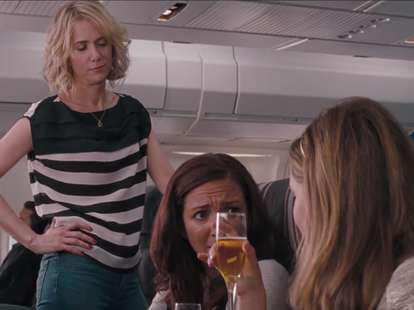In a lively scene from the movie "Bridesmaids," the image captures an airplane setting, likely in first-class due to the spacious two-seat arrangement. Seated and engaging in conversation are two women in white tops, each holding a glass of champagne. The woman closer to the camera has lighter brown hair, while her companion has darker brown hair. Positioned in the aisle, Kristen Wiig's character, with medium-length curly blonde hair, stands dramatically. Dressed in blue jeans and a distinctive smock sweater with black and white thick stripes, she has a necklace that adds to her look. With one hand assertively placed on her hip and the other on the back of a seat, she sports a perturbed and slightly smug expression, possibly due to being ignored by the seated women. Her eyes are somewhat closed, suggesting a hint of exasperation. Overhead compartments illuminate the scene with bright daytime light, highlighting the tension and humor in this memorable movie moment.